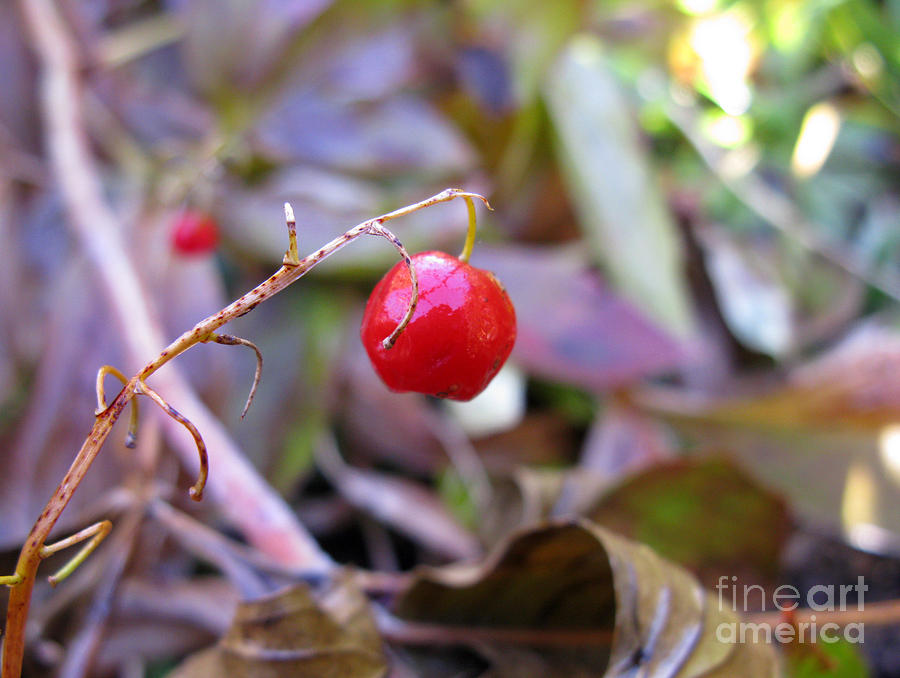This highly detailed, professional close-up photograph captures a vibrant, bright red cherry hanging from a thin, yellowish-brown vine. The cherry, gleaming with ripeness, dominates the foreground, attached to a delicate branch. The image showcases the cherry in exquisite detail, highlighting its smooth texture and rich color, forming the central focus of the composition. Behind it, slightly blurred, is another cherry, providing depth and a sense of continuity. The background, while intentionally out of focus, reveals the presence of large leaves and assorted vegetation, suggesting the setting might be a garden or natural environment. The weight of the cherry gently bends the slender vine, further emphasizing its ripeness. The photo, marked with a watermark in white text reading "Fine Art America" in the lower right corner, embodies the essence of fine art photography, combining natural beauty with artistic presentation.